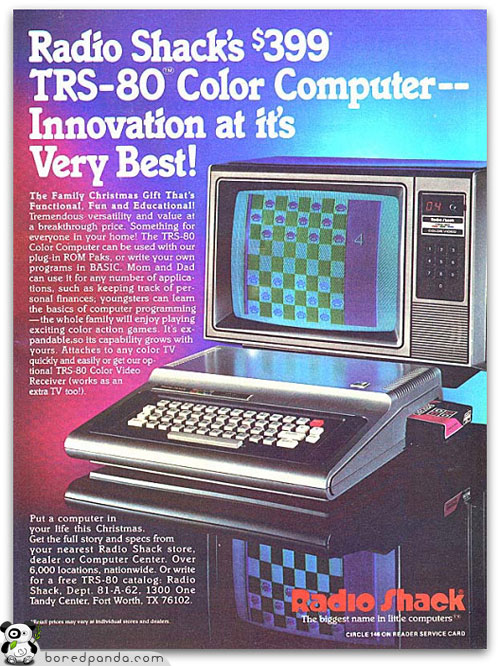The image is a vibrant and colorful poster advertising the RadioShack TRS-80 Color Computer, available for $399. It exudes an unmistakable 80s aesthetic with a striking color scheme featuring shades of purple, pink, red, dark blue, light blue, black, and green. The poster prominently showcases the computer, which resembles a small CRT TV. The monitor displays a checkers game in green, purple, and white, underscoring the product's recreational as well as educational purpose. 

The computer itself features a typewriter-like keyboard with predominantly white keys and a single, conspicuous red key in the top right corner. Additionally, there is a keypad on the right side of the monitor with numbers ranging from 1 to 9 and 0. A pink and black cartridge is visible inserted into the side of the computer. The poster highlights the tagline "Innovation at its very best" and pitches the TRS-80 as an ideal family Christmas gift that is functional, fun, and educational, emphasizing its versatility and value. The ad encourages consumers to learn more about this breakthrough product at any RadioShack store, dealer, or computer center, boasting over 6,000 locations nationwide. The lower portion of the poster includes the RadioShack slogan "The biggest name in little computers," and the watermark "boardpanda.com" is visible in the bottom left corner.